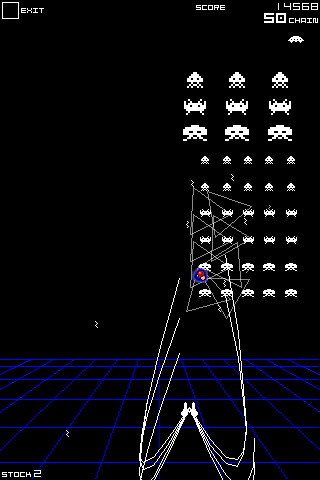The image is a detailed screenshot of a classic-style Space Invaders video game. The background is entirely black, highlighting the cobalt blue grid that forms the floor at the bottom half of the screen. On the bottom left corner, the text "Stock 2" is written in white font. The upper left corner features a white square with the word "exit" written to its right. The scoring details are prominently displayed with "score" written near the top right, followed by the numbers "14,568" and a "50 chain" indicator beneath it. The right side of the screen hosts various white alien figures resembling those from Space Invaders, with a mix of larger aliens arranged in a three-by-three grid at the top and smaller aliens below in six rows of five. Additionally, there are complex, scribbled lines extending from a main spaceship at the bottom left, curving upwards and towards the aliens, with a colorful concentric circle over one of the aliens on the far left of the second row.